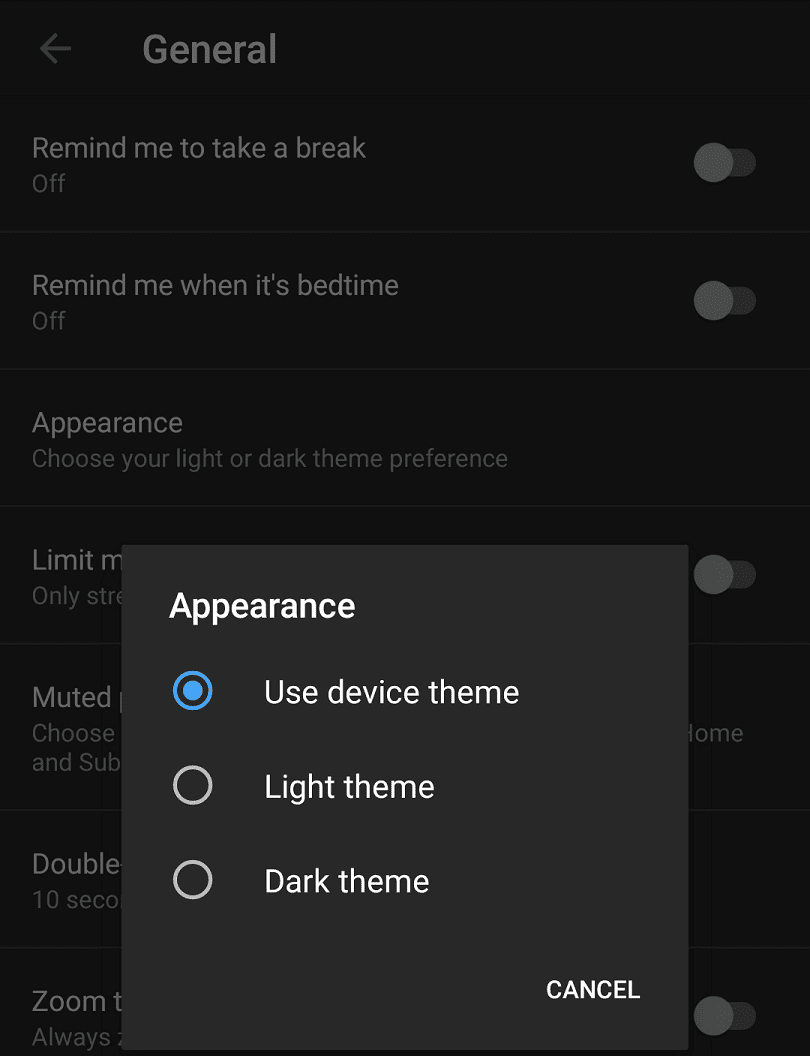This image is a cropped screenshot of the 'General Settings' tab within an app, displayed in night mode on a mobile device. The background is solid black to reflect the night mode theme of the phone. At the top left corner, the word "General" is prominently displayed in large white letters. To the left of this heading is a left-facing arrow icon, likely used for navigation.

Under the heading, there is a vertical list of settings options. The first option, "Remind me to take a break," is accompanied by a toggle switch on the right side, which is currently turned off. Below it, the second option is "Remind me when it is bedtime," also with a toggle switch that is off.

Further down is the "Appearance" setting, which allows the user to select their preferred theme mode - light or dark. Beneath this setting, there is a popup box showing three choices: "Use device theme," "Light theme," and "Dark theme." The default selection, "Use device theme," is currently enabled, and since the phone is in night mode, the app's appearance is also in night mode.

Although partially obscured by the popup box, four additional settings options are visible at the bottom of the list.